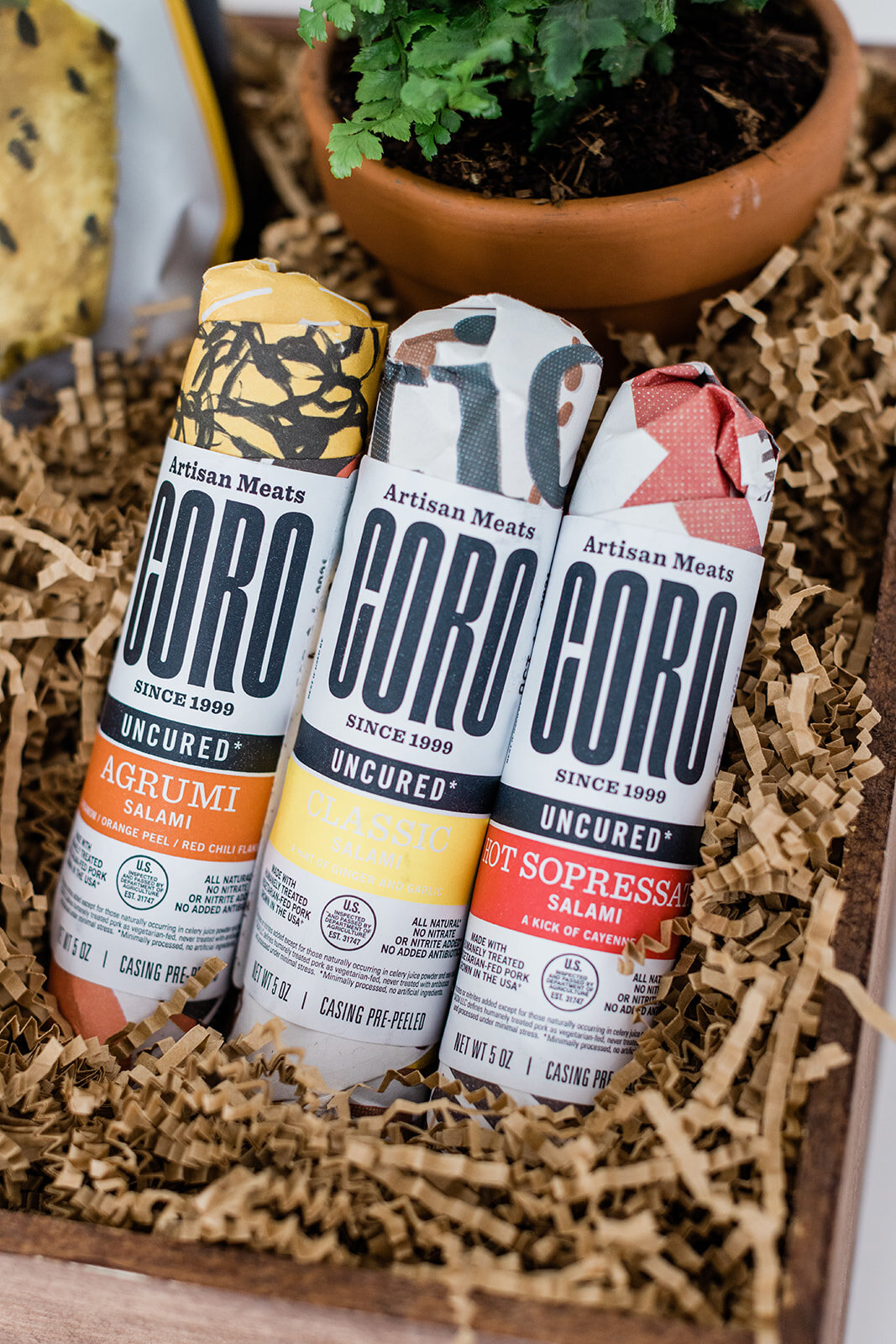The rectangular image, taller than it is wide, features a brown wooden gift box filled with finely shredded, crinkly brown paper, resembling Easter grass but made of a cardboard bag material. Nestled amid the filler are three tubes of salami from Artisan Meats, branded as Coro since 1999, each with colorful and funky designs. The salami varieties include one labeled "agrumi salami," another "hot sopressa salami," and a third logo with a yellow banner whose white writing is not clearly readable. The labels indicate the meats are uncured and nitrate-free, weighing approximately five ounces each. At the top of the image, part of an orange flower pot with an indeterminate white and yellow object in the top left corner is visible.